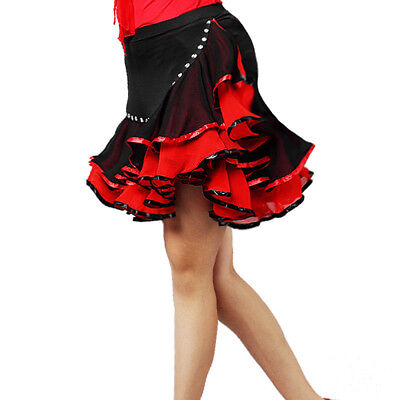The image showcases the lower half of a female wearing a striking dress with a white background. The dress, which has a flamenco-inspired design, features a bright red blouse seamlessly transitioning into a high-waisted black skirt. The skirt is layered and puffy, flaring out elegantly above the knees. The black top section of the skirt boasts intricate red underlayers, giving it a bell-like silhouette and dynamic movement. The dress also has subtle black highlights and small circular patterns adding to its intricate design. The image captures the woman from her waist down to her ankles, with her feet not shown, presenting an evocative snapshot of vibrant Latin American-inspired fashion likely suited for a night out or dancing event.